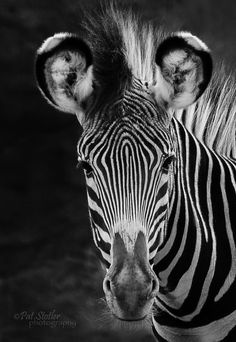In this striking black and white portrait, a zebra stands front and center, captivating viewers with its direct gaze. The zebra occupies the middle to the right side of the image, its expressive, rounded ears prominently displayed with black tips contrasting against a mix of white and black fur. Its face and part of its neck are clearly visible, with a distinctive mane starting from the head and continuing down the spine. The zebra's iconic stripes start narrowly at the front of its face and gradually widen as they progress towards the neck, enhancing the animal’s majestic appearance. The background is predominantly black with subtle grey tones, adding depth to the composition. In the lower left corner, the photographer's credit reads "Pat Stotler, photographing."